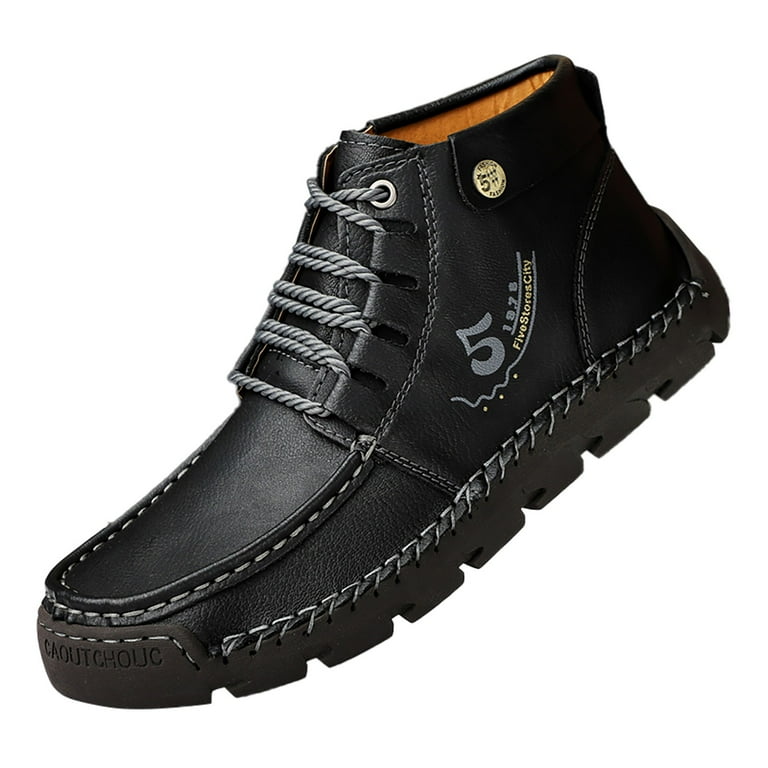This single photograph showcases a black leather ankle-length boot with intricate detailing. The exterior of the boot is constructed from high-quality black leather, accented with gray stitching. The boot features gray and black striped braided laces and a circular golden button on the top outer side. Notably, the left side of the boot is adorned with the number "5" in bold, along with the text "5 Store City, 1978" in yellow letters. The interior of the boot is lined with a light brown or yellow-orange fabric, visible from the top view. The sole, made of black rubber, displays large treads and is inscribed with "C-A-O-U-T-C-H-O-L-I-C" on the front. Despite the premium materials, the overall design leans more toward a casual style rather than formal.